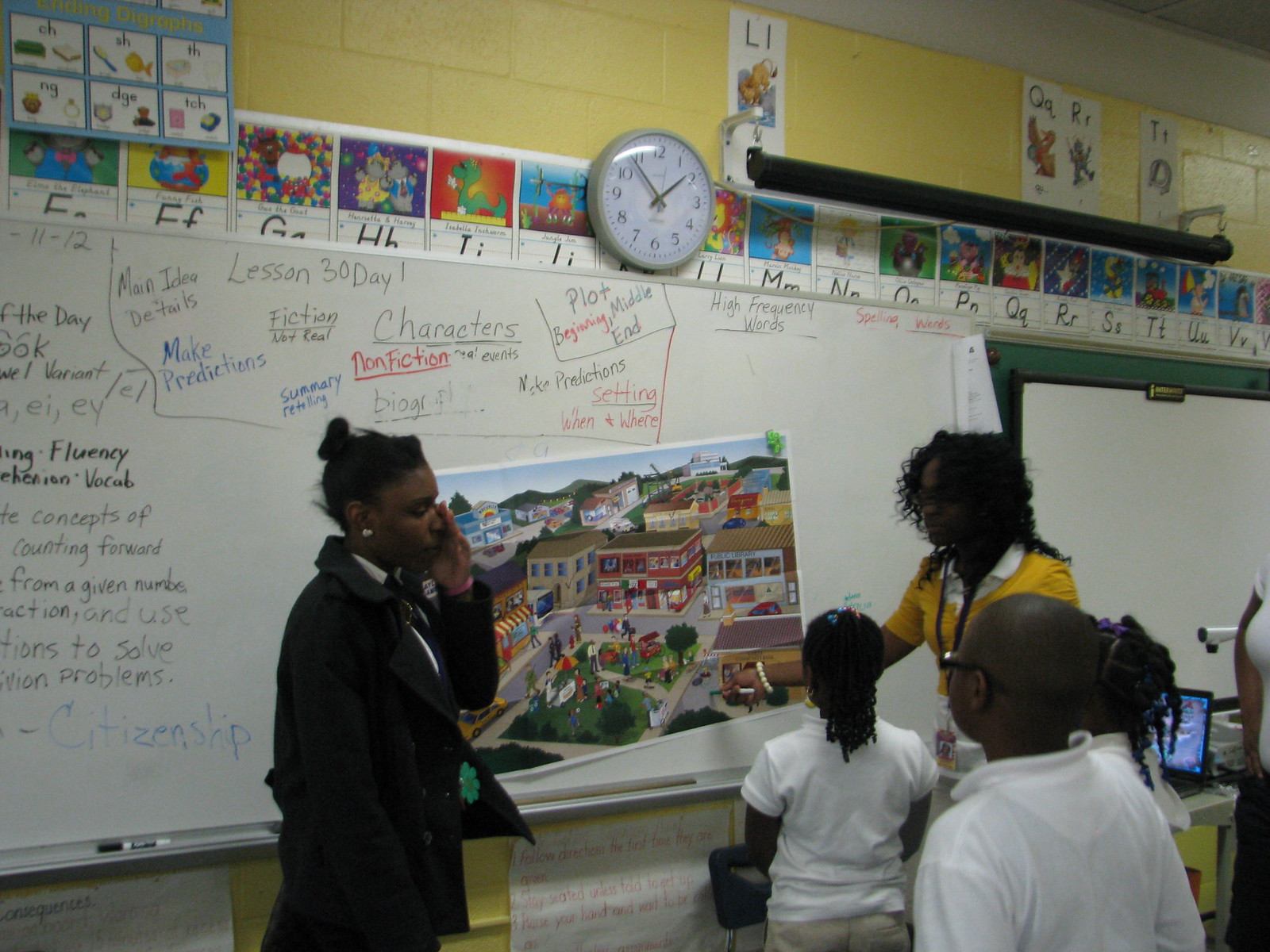In the classroom, a learning session unfolds with a blend of attentive and engaging energies. The whiteboard, filled with various lessons and notes, serves as the focal point where a city map graphic captures the students' attention. Positioned around the whiteboard, the students are diligently standing and gazing at the instructive map. Two black women, the main teacher in yellow with a hint of white underneath, and a teacher's assistant on the left in a black jacket with white accents, supervise the session. Despite their collaborative effort, the assistant appears slightly frustrated or disappointed, her hands on her face displaying her emotions clearly. The classroom, adorned with an alphabet display at the top, resonates a vibrant mix of colors—yellow, red, green, blue, white, black, light blue, and orange. Though the exact time reads 1:53 on a wall clock, the ambiance makes it difficult to discern whether it's daytime or nighttime. This scene was captured from behind, showing the involved interaction among the educators and the young students, who are neatly dressed in white with their hair tied up.